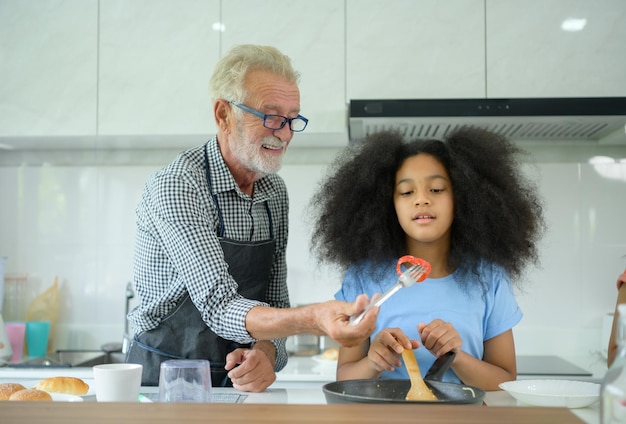In a bright, clean kitchen, an elderly white man with white hair, a white beard, and blue-framed glasses is teaching a young light-skinned, mixed-race girl, around 13 years old, how to cook. The man, who is smiling, has a wrinkled face and wears a blue and white checkered shirt paired with a black apron. He holds a fork with a piece of red bell pepper on it, offering it to the girl. The girl, with natural hair styled in two side ponytails, wears a light blue t-shirt. She stands next to a stove, holding a wooden spoon over a skillet, looking intently at the bell pepper. Around them on the counter, there are various kitchen items, including a pink and teal cup, an empty bowl, an upside-down Tupperware, a few small biscuits, a piece of bread, and a white cap. The scene captures a moment of shared learning and concentration.